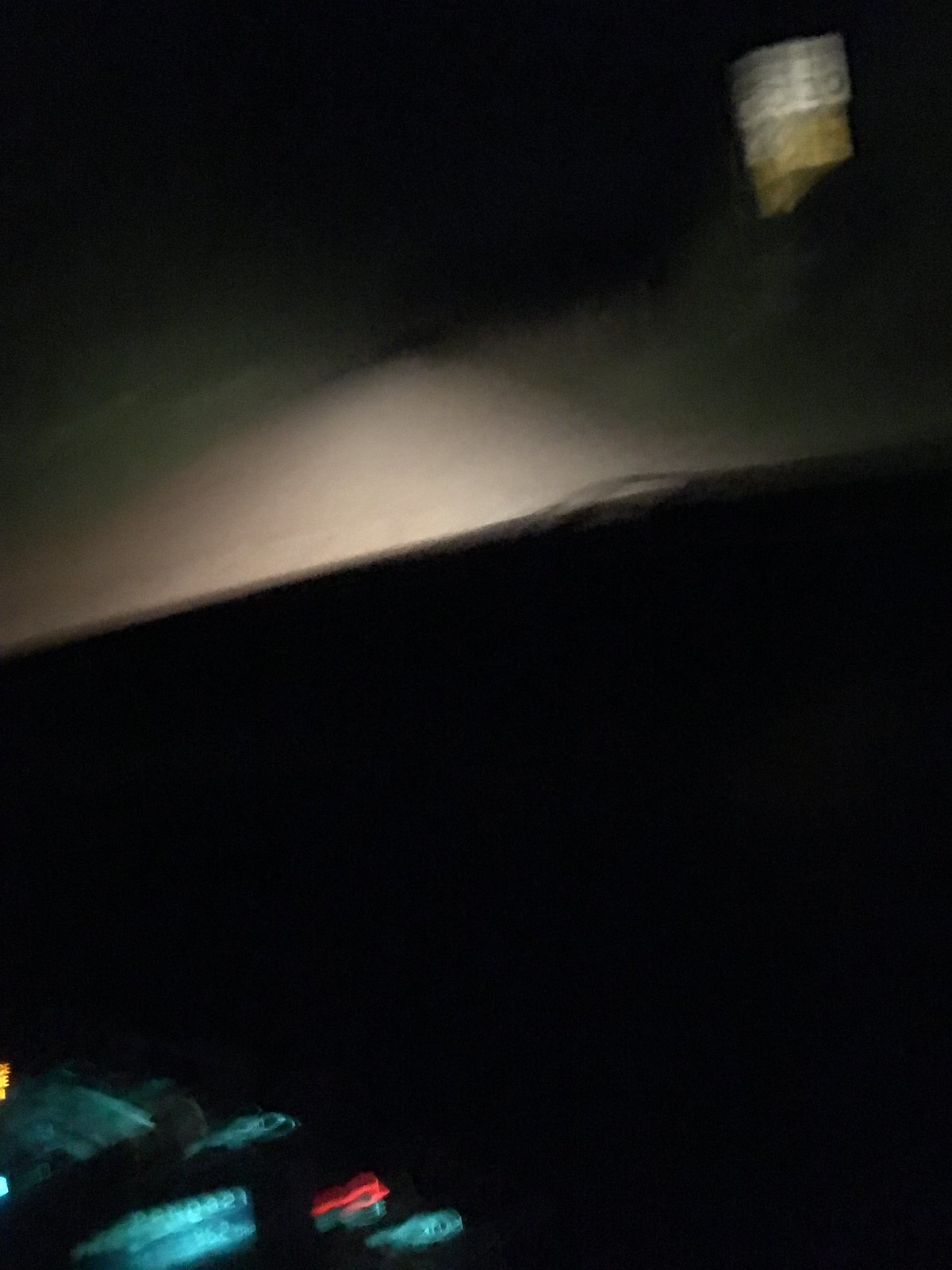This is a dark, extremely blurry photograph taken from inside a moving car at night. The dirt road ahead is illuminated only by the car's headlights, creating a narrow view framed by motion blur. The road itself is flanked by hints of green foliage, adding depth to the night scene. The dashboard is dimly lit by the car's interior lights, including blue and red hues from the center console controls such as the radio and AC buttons. A speed limit sign reading "30" is visible but fuzzy to the right side of the image. Stray marks in blue, green, and red from the interior lights and motion cuts across the image, adding to the overall blur. In the upper right corner, there's a blurred white and gold square, possibly part of the car's interior or something reflective along the roadside, and silhouettes of trees can be discerned in the surrounding darkness, blending with the black sky.